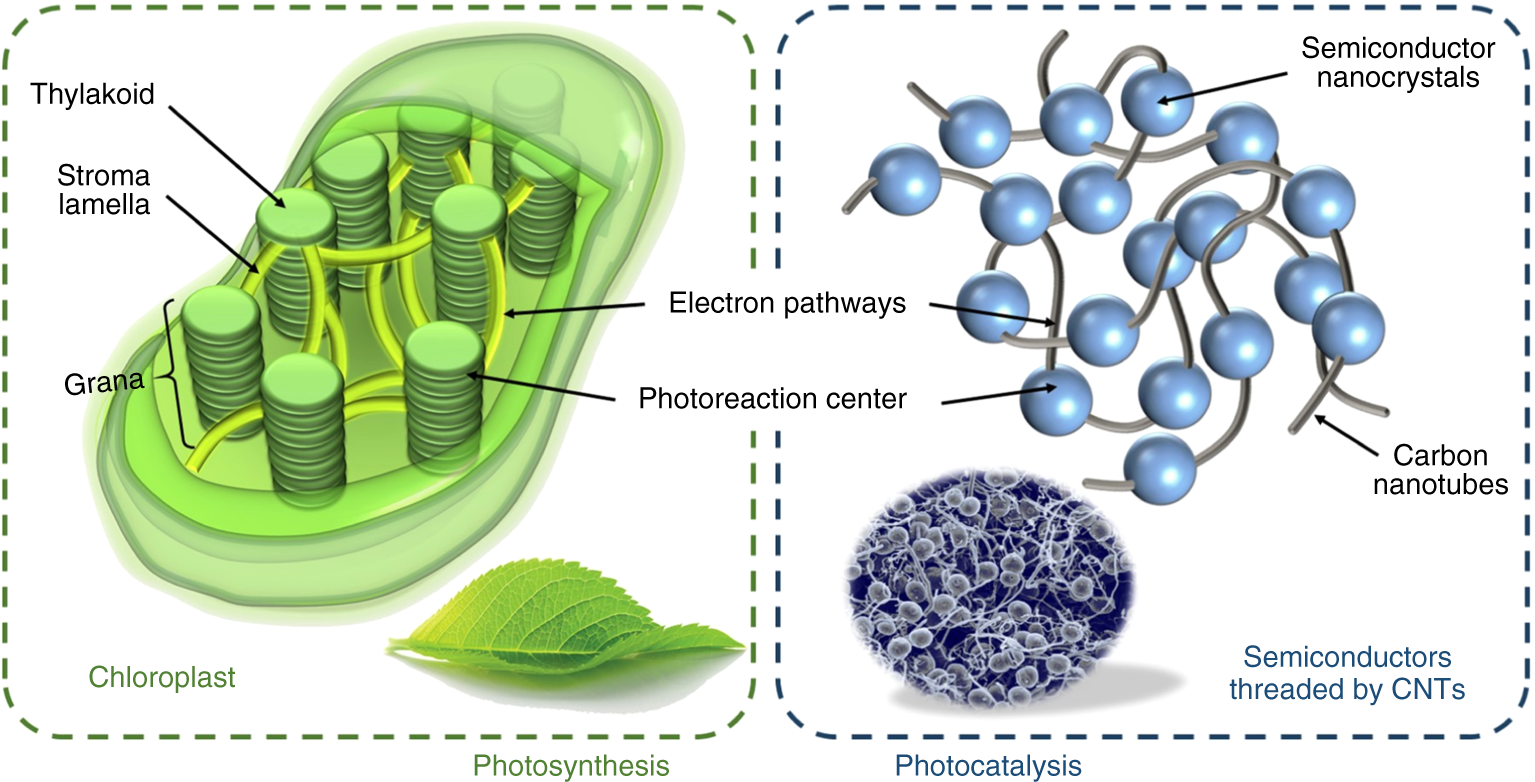The image is an educational infographic presented in a cartoon style, illustrating two distinct processes side-by-side. The left side, encased in a dashed green border, is centered around the concept of photosynthesis. It features a cutaway diagram of a chloroplast, highlighting various components such as thylakoid, stroma, lamella, and grana. These components are depicted as stacked green circles connected by pathways, all confined within a dotted green square. At the bottom of this section, a label reads "Photosynthesis."

The right side of the infographic, outlined with a dashed blue border, delves into photocatalysis. It showcases interconnected blue circles, resembling berries, which represent semiconductor nanocrystals and carbon nanotubes (CNTs). Labels identify "semiconductors threaded by CNTs" and "electron pathways," all within a dotted blue square. The bottom of this section is marked with the label "Photocatalysis." The infographic effectively juxtaposes the two processes, using analogous visual structures and detailed labeling to enhance educational clarity.